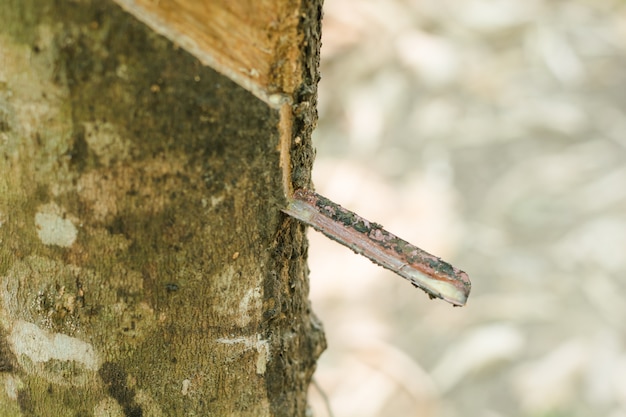This close-up image captures the detailed texture of a tree trunk. The trunk, positioned on the left side of the frame, displays a patchwork of mossy, brown bark interspersed with white, pinkish-red, and darker spots. There are grooves and indentations on the bark, one of which is leaking white liquid into a wooden spout. This spout, fashioned from a rectangular piece of bark that has peeled off and juts out at a right angle, channels the liquid towards the tip. This rectangular bark piece, about three inches long, appears to have been dislodged by a combination of gravity and possible decay or disease, revealing the lighter, inner layers of the tree just above it. The right side of the image is blurry and out-of-focus, rendering the background as a mix of gray, white, and faint greenish hues, possibly indicating foliage or sky, but remaining indistinct and abstract.